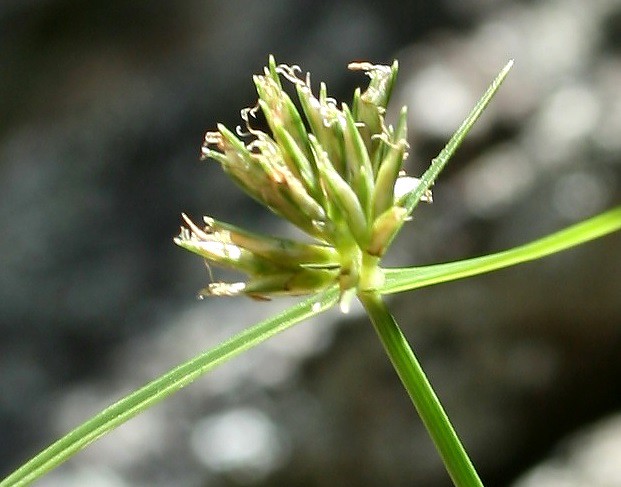This color photograph captures a single plant as the focal point, set against a blurred and indistinct black-and-white background, likely taken outside during a sunny morning or shortly after a rainstorm. The plant, prominently centered, features a long green stem that rises from the bottom right of the image. It has two outstretched leaves resembling arms, each adorned with tiny droplets that could be morning dew or remnants of recent rain. At the top of the stem, there are multiple small buds that are partially opened, showcasing a slight transition into delicate white flowers. The green of the plant is vibrant near the leaves and stem but gradually fades to a softer hue towards the budding tips. Despite the background appearing rocky, dry, and sunlit, the primary focus is squarely on the intricate details of this striking plant in the midst of its blooming process.